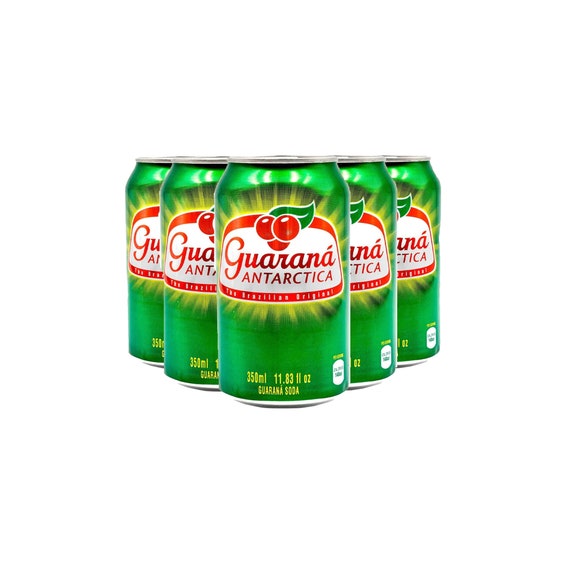This detailed color photograph depicts a neatly arranged triangular formation of six green aluminum cans. The cans are set against a plain white background. Each can prominently features a white section bordered in red at the top, displaying three overlapping red cherries with a green leaf, all outlined in white. Below this emblem, the text "Guarana Antarctica" is written in bold red script. The cans are labeled as guarana soda, with a capacity of 350 milliliters (11.83 fluid ounces). Amidst the predominantly green design, there is yellow text at the bottom providing additional details. This meticulous arrangement showcases a European beverage known as Guarana Antarctica.